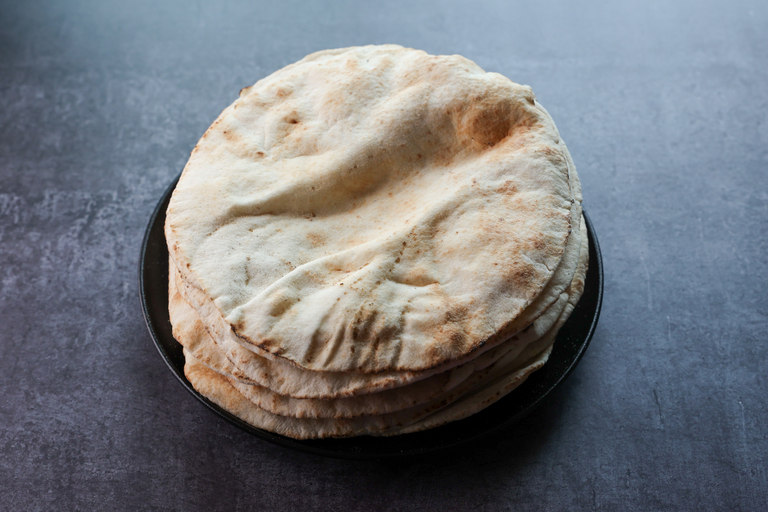The image showcases a stack of homemade pita bread, prominently displayed on a black plate or bowl. The photo, taken from a top-down perspective, reveals a neatly piled arrangement of roughly six pieces of pita, centered against a slightly darker slate gray or charcoal blue background. Each piece of pita features the typical light off-white to light brown hues, with darker medium brown spots and edges that suggest crispiness. The top pita is notably wrinkled with two distinct folds, giving it a unique texture and a slightly plump appearance. The overall lighting of the scene emphasizes the fresh and appetizing nature of the bread, enhancing the details of the soft, malleable surface and subtle air bubbles. The minimalist background draws attention solely to the stack of pita bread, making it the indisputable focal point of the image.